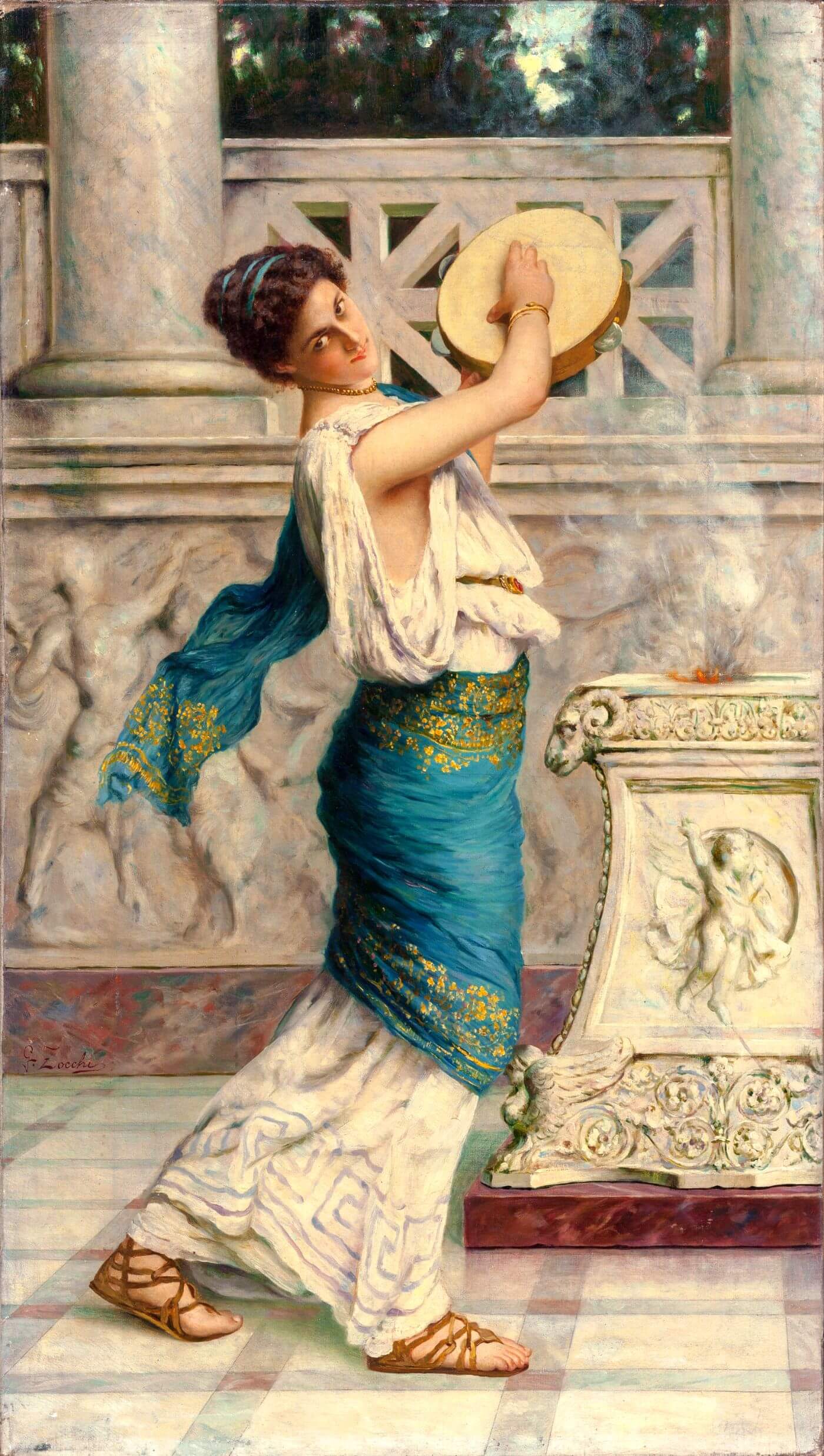The painting depicts a woman from ancient times, positioned centrally in a vertical, rectangular frame. She is draped in a long, white sleeveless gown with flowing folds, extending from her ankles to her shoulders. Wrapped around her waist is a blue scarf adorned with gold emblems, which flows over her shoulder and trails behind her. She wears brown sandals with straps. Her head is adorned with a blue headband, holding back her brown hair. The woman is standing next to the base of a statue, though the object atop the base is indiscernible. She holds a tan-brown tambourine in one hand, poised as if ready to play it. Her posture faces to the right, with her head turned over her right shoulder. The backdrop features ornate Roman or Greek pillars in a purplish cream hue, with glimpses of dark green tree leaves and a blue sky. The environment suggests an ornate, classical setting that contrasts sharply with her simple, yet elegant attire.